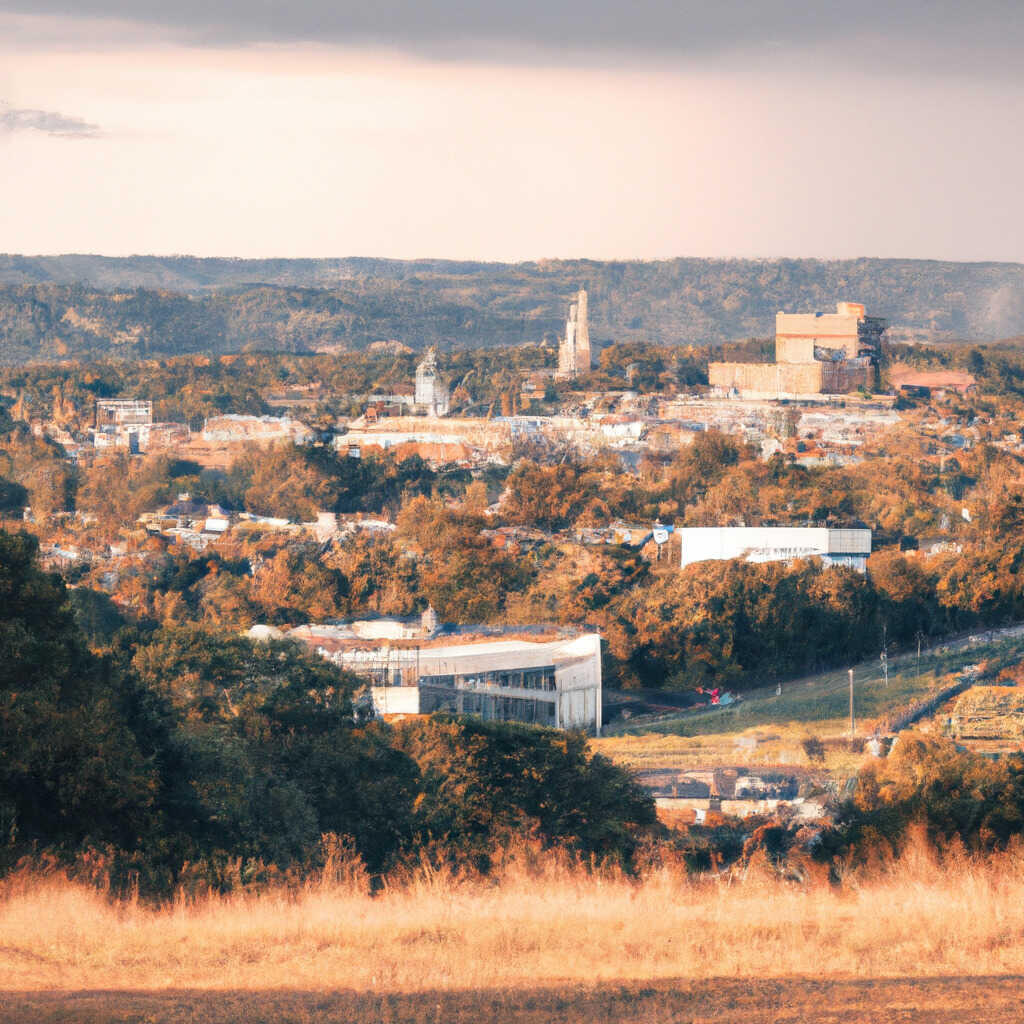This large square painting captures a breathtaking landscape viewed from atop a hill. In the foreground, tall, brown grass suggests a seasonal shift, possibly autumn. Just beyond this is a dense section of green foliage, featuring a mix of bushes and trees. The scene then slopes down into a valley where a winding road appears off in the middle distance, flanked by more grassy areas and patches of trees. 

To the middle left stands a building, with more scattered structures of varying sizes in the background—some tan, some white, suggesting a rural setting rather than an urban one. Among these structures, a prominent white, circular building with numerous windows stands out. Further back, more buildings emerge, including some taller ones and even a few skyscrapers, which eventually give way to a mountainous backdrop. 

The sky overhead is layered in a gradient of colors, starting with a gray hue at the top and transitioning to a yellowish-pink near the horizon, adding to the painting's serene yet complex atmosphere.